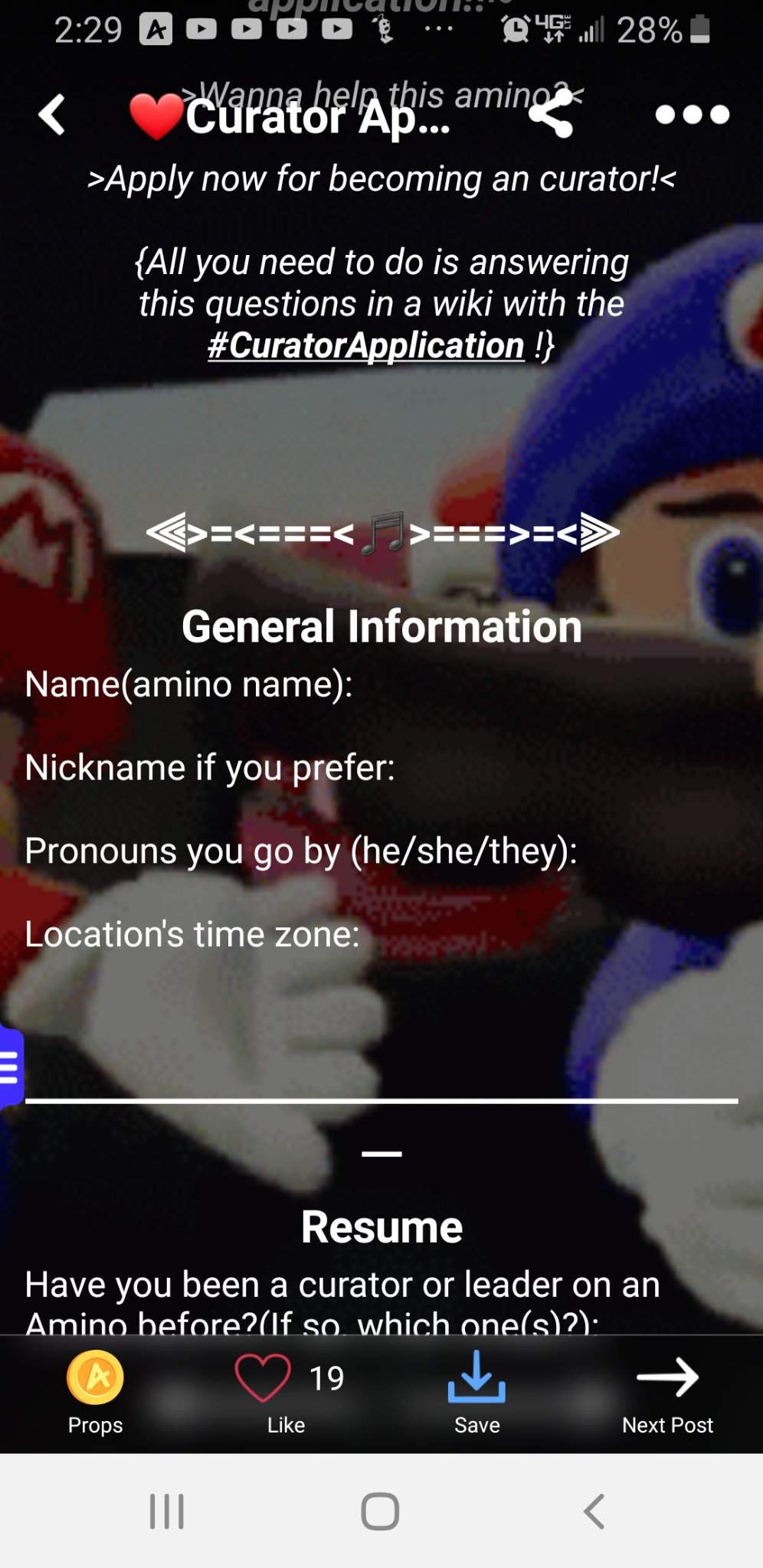Screenshot of Mobile Phone Display Featuring Super Mario Game and Application Details

This screenshot, captured on a mobile phone oriented vertically, features a dark background and various interface elements. The top left-hand corner of the screen displays the time as 2:29, while the top right-hand corner shows the battery level at 28% and indicates a 4G network connection. At the very top, a series of small YouTube video icons are visible against a gray background.

The main image appears to be a screenshot from a Super Mario game. On the left side, Mario, identifiable by his iconic red cap and white-gloved hand, is prominently featured. On the right side, there appears to be another version of Mario, distinguishable by a blue hat, large blue eyes, and white gloves. Both characters seem to be inside a vehicle.

Overlaying this background is a block of white text. At the top, there is a small red heart icon followed by the text "curator AP...". Below it, the text reads: "Apply now for becoming a curator. All you need to do is answer these questions in a wiki with the hashtag #curator application."

Further down, there are decorative arrows made up of equal signs and greater-than/less-than symbols pointing left and right, with a musical note icon in between. This section is followed by more white text titled "General Information," listing the requirements:
- Name (Amino name, nickname if you prefer)
- Pronouns you go by (he, she, they)
- Location (time zone)

The final section of the overlay text inquires about previous experience: "Have you been a curator or leader on an Amino before? If so, which ones?"